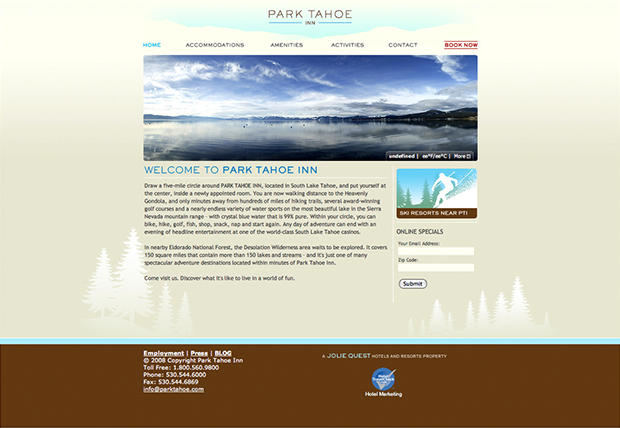Welcome to Park Tahoe Inn

The picturesque image showcases the tranquil beauty of Park Tahoe Inn. At the forefront lies a vast, serene lake, with majestic mountains and dense trees in the background. A veil of white fog hovers over the lake, adding a mystical charm to the scenery. Above, the sky is a brilliant blue adorned with some fluffy clouds. To the right, there is an animated silhouette of a skier gliding down a hill, flanked by green trees, representing the various recreational activities available. The webpage features a beige color palette with white tree accents, a light blue dividing line, and a brown bottom section. Important information such as accommodations, amenities, activities, and booking options are prominently displayed. Highlights include online specials and submission options. At the bottom, the text reads "Environment, Prices, Blob 2008 Corporation, Park Tahoe Inn," and the hotel is marketed by Joe Gulley Quest. A distinctive blue circle with a white triangle, resembling a cocktail cup with a toothpick, adds a unique logo to the page.

Book now to experience the serene beauty and engaging activities at Park Tahoe Inn!